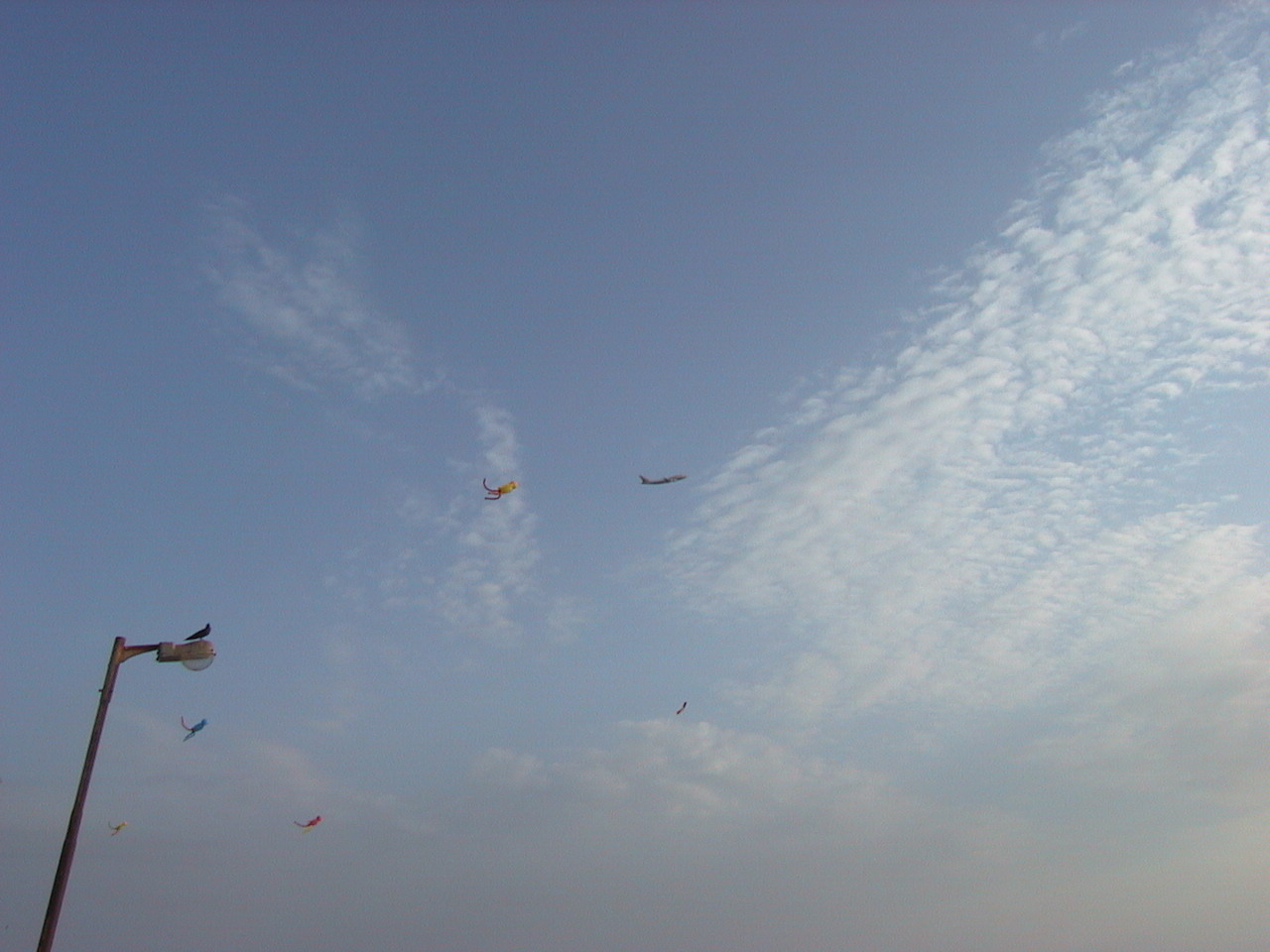The photo captures a vibrant sky scene filled with interesting elements. From the ground looking upward, the predominantly blue sky is scattered with thin, wispy clouds that resemble scales or starting to drift apart. In the very center of the image, a tiny passenger plane is visible, dwarfed by the vast sky around it. Flying in the foreground are several vibrant windsock-type kites, each trailing streamers. Directly behind the plane is a distinctive kite with a long tubular yellow top and trailing streamers, giving a whimsical illusion of chasing the plane. In the lower-left corner, three additional windsock kites—one blue, one yellow, and one red—are clustered together, their shapes and streamers clearly visible despite their distance. A nearby light pole with a glass fixture rises from the bottom left corner of the frame, crowned by a dark bird perched on top, possibly a crow or a gull, providing a touch of life and grounding to the otherwise skyward scene.